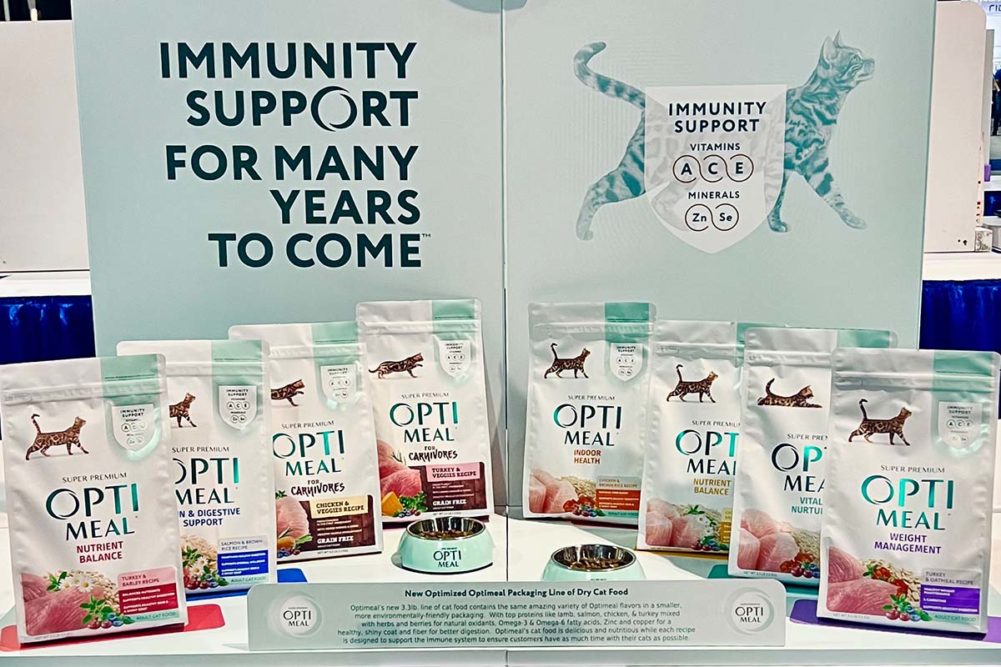The advertisement display features eight bags of OptiMeal cat food, meticulously lined up on a counter. Each bag prominently showcases the brand name 'OptiMeal' centered in large letters, with various specific nutritional benefits highlighted underneath such as Nutrient Balance, Digestive Support, Carnivores, Indoor Health, Vital Nutrients, and Weight Management. Each bag also depicts a cat—either standing, walking, or sitting—displaying different breeds and poses. The bags are predominantly white with colored bottoms that indicate the ingredients contained within.

Behind the bags, a poster board in light aqua green displays a headline reading "Immunity Support for Many Years to Come," accompanied by a picture of a cat tinted in aqua hues and wearing a shield symbolizing immunity support. Additional nutritional details listed include vitamins A, C, E, and minerals zinc (Zn) and selenium (Se). The display also features two turquoise-colored pet food dishes. Each OptiMeal variety is designed to cater to specific dietary needs, ensuring comprehensive health support for cats.